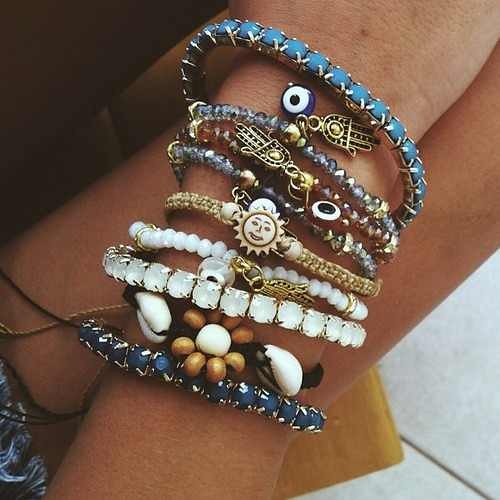In this close-up color photograph, we see a detailed view of a person's two arms adorned with an eclectic mix of beaded bracelets. The upper arm stretches diagonally from the bottom left to the upper right corner, showcasing a vivid array of nine bracelets in various styles and colors. Among these, there are several blue beaded bracelets, one featuring an eye trinket and another with a small figure. A striking white and beige bracelet is adorned with a large beaded flower. A shimmering bracelet appears to be crafted from white diamonds, complemented by another embedded with white pearls. Prominent is a gold bracelet with a central sun emblem, adding a unique charm to the ensemble. Additionally, there are teal bracelets stitched with white thread and a brown bracelet. Some bracelets are further embellished with charms, including a palm hand and shells. The background shows a beige wooden surface and a piece of fabric, likely worn by the person, in blue with lighter blue and white designs. The lower left corner reveals a grey-tiled flooring with a distinctive diagonal line.